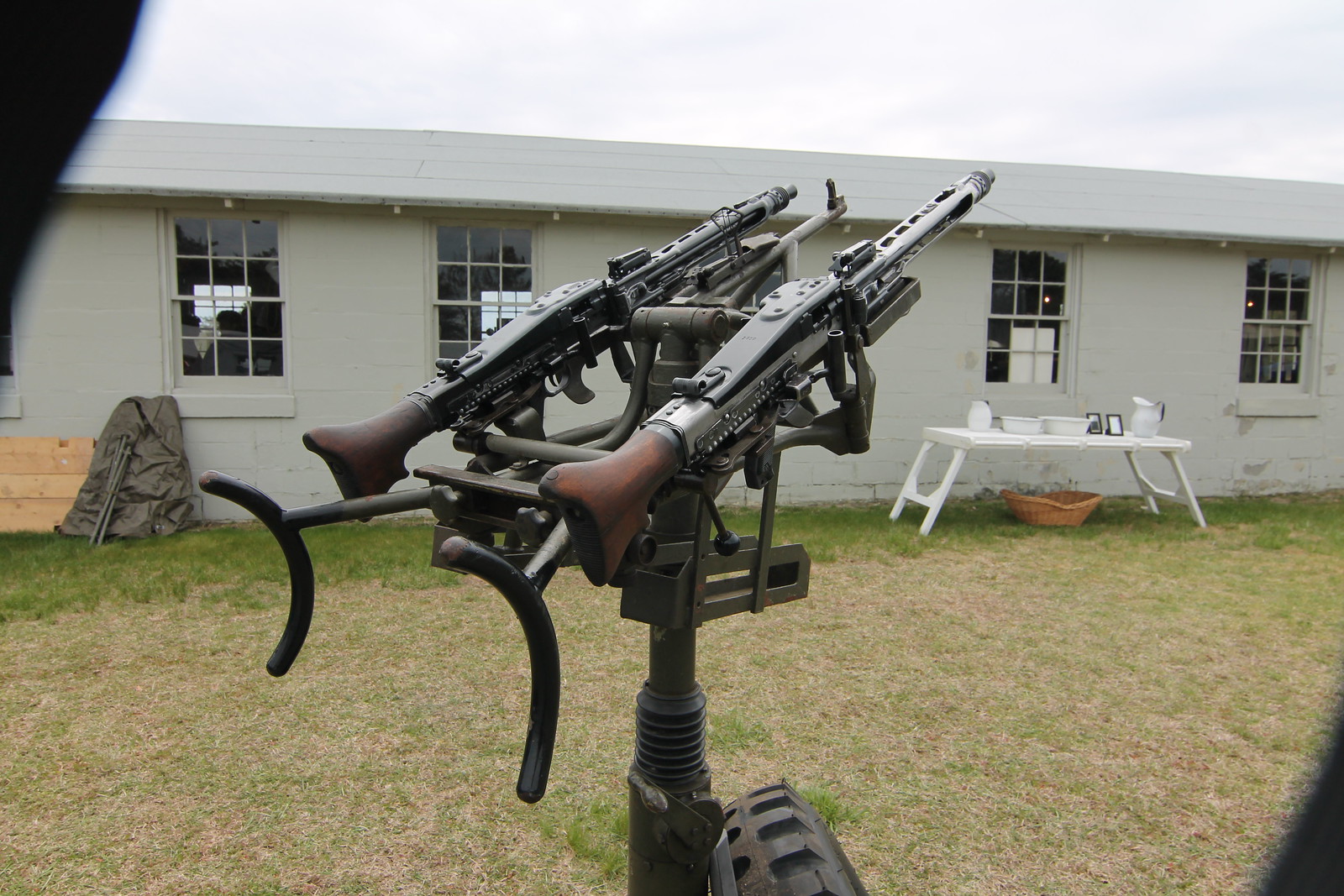In this outdoor color photo, likely taken with a cell phone, we see a detailed setup of two long guns mounted on a black stand. The scene is set in a grassy field next to a long white building with multiple windows, suggesting a military practice range or shooting training ground. The guns, which resemble heavy machine guns or possible anti-aircraft weapons, feature thick barrels and wooden stocks, hinting at a large caliber of ammunition. Each gun appears to be partially exposed, showing various bolts and internal parts, leading to speculation that they might be incomplete or under construction. The stand is grounded with a substantial base, possibly for stability during firing, and the overall setup gives an impression of a military apparatus designed for rapid, mounted firing, akin to weapons used on tanks or other military vehicles. The surroundings and the lack of text on the image further emphasize the typical military training environment.